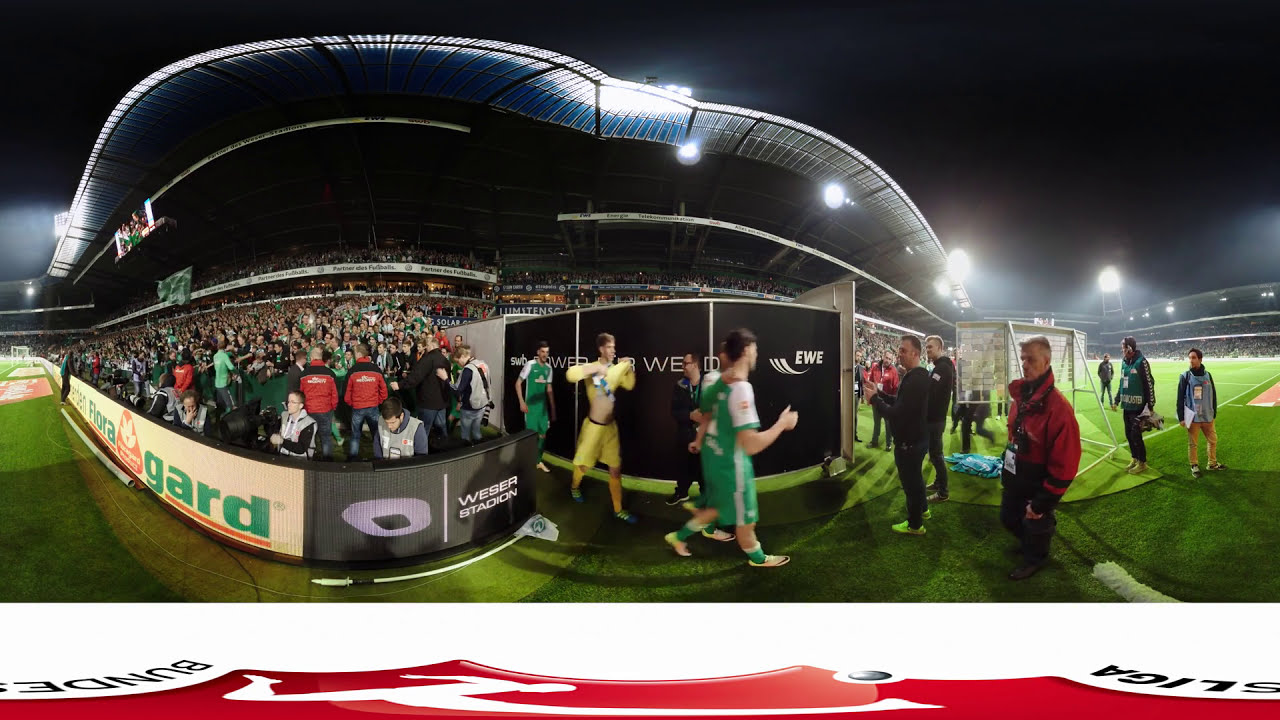The image is a panoramic, seemingly fisheye, shot taken at a soccer stadium at night. The sky is dark, contrasting with the bright illumination from the stadium lights. The left portion of the image displays a densely packed crowd of spectators in the stands, partly sheltered by the stadium's roof, which extends to the middle-right of the image. Below this crowd, there is a short wall with black advertisements. To their right, a group of players in green and yellow uniforms are emerging from a tunnel or gate, with advertisements and netting visible around them.

Among the players, one in a yellow uniform is depicted taking off his shirt. Adjacent to these players stands a group of individuals in black and red coats, likely coaches and photographers, facing the players. These individuals are wearing badges and lanyards, with some holding notebooks. The stands in the background are full of spectators, with bright lights on top, contributing to the well-lit scene.

The right side of the image captures more people standing on the grass, along with another distant set of stands and stadium lights. The field is a vivid green, and the use of a panoramic lens creates a curved distortion affecting the barrier between the crowd and the field. Finally, the image is bordered by a thick white frame at the bottom, featuring a red and white banner with upside-down black text on both sides.